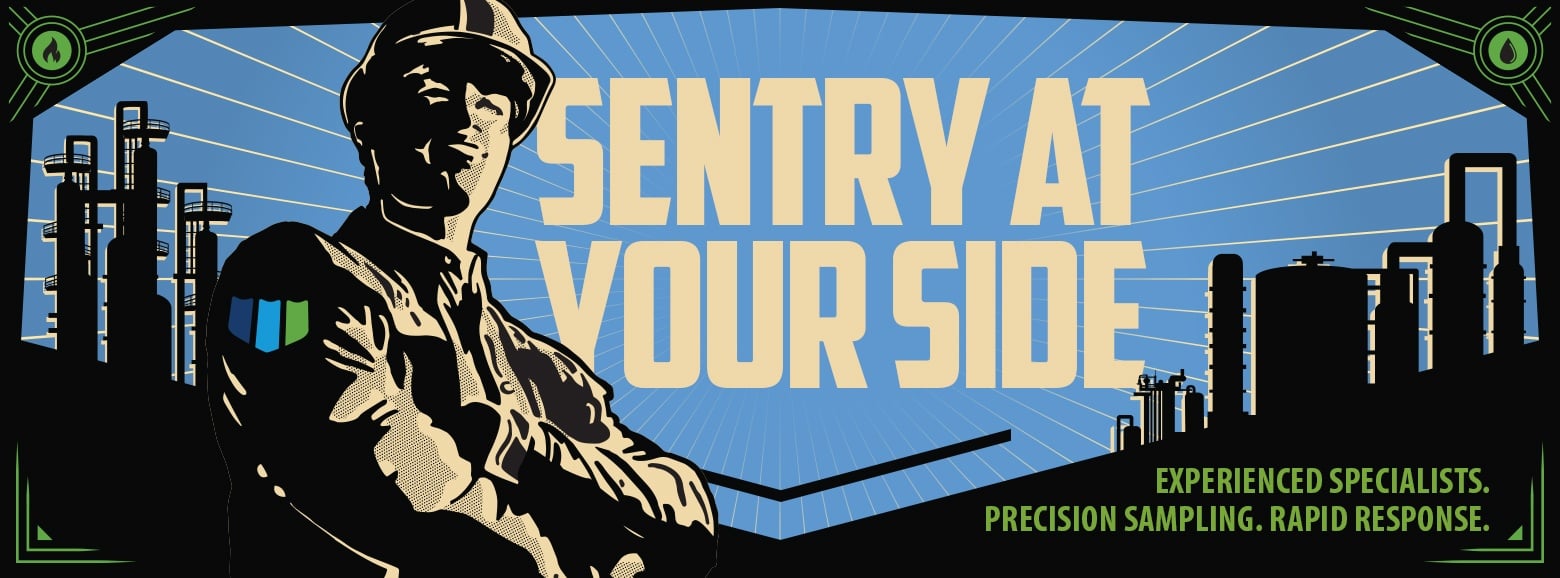The image is a vertically oriented banner, primarily designed as an advertisement, featuring a combination of detailed graphics and text. The background is predominantly black with green geometric shapes in the corners, such as circles and angles, adding a sense of design complexity. In the top corners, a logo appears within green circles—one resembling fire and the other a water drop, emitting lines outward that simulate sun rays. At the center of the banner, large, bold, light yellow text reads, "Century at your side," serving as the headline. 

On the left side of the banner, there is a shaded outline of a man, possibly a soldier or worker, dressed in a uniform that includes a helmet and a badge on his sleeve, with his arms folded across his chest. The man's face is visible but lacks detailed features like eyes, giving it a grayish-black hue. Behind this figure, a cityscape is depicted, including buildings and towers that could be construed as machinery or other industrial structures. Accompanying this visual, additional green text at the center and bottom right of the image states, "Experience, Specialist, Precision Sampling, Rapid Response."

Overall, the banner blends elements of illustration and text to create an engaging advertisement, possibly intended for a company or organization's website.